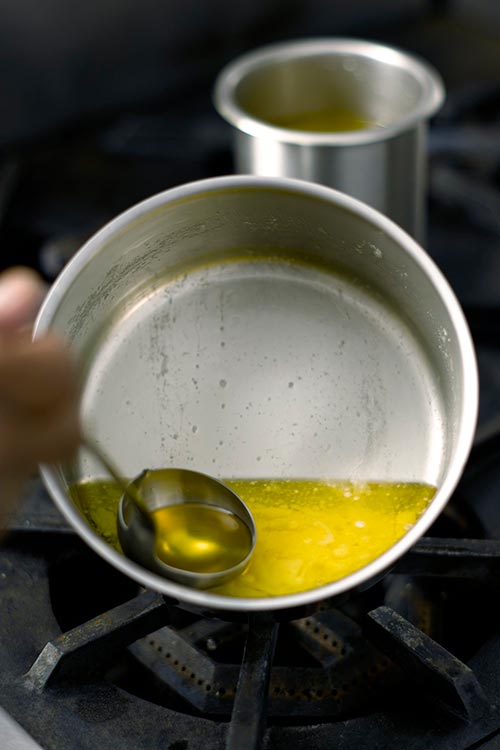The high-definition image, likely taken by a food blogger, presents an intricate culinary scene set in a dimly lit kitchen. At the forefront, a round silver pot, placed on a gas burner with distinctive black metal arms, contains a vivid yellow liquid that resembles melted butter or possibly oil. This yellow liquid, swirled and slightly bubbly, fills the bottom of the pot and leaves streaks along its upper edges. A blurred hand is seen holding a large, silver metal ladle, which is partially submerged into this liquid, capturing it within the spoon. In the background, there's a second tall silver pot with a faint yellow tint, indicating it may contain a similar substance. The background remains intentionally blurred, drawing focus to the detailed textures and colors of the liquid in the pot and the surrounding metallic elements.